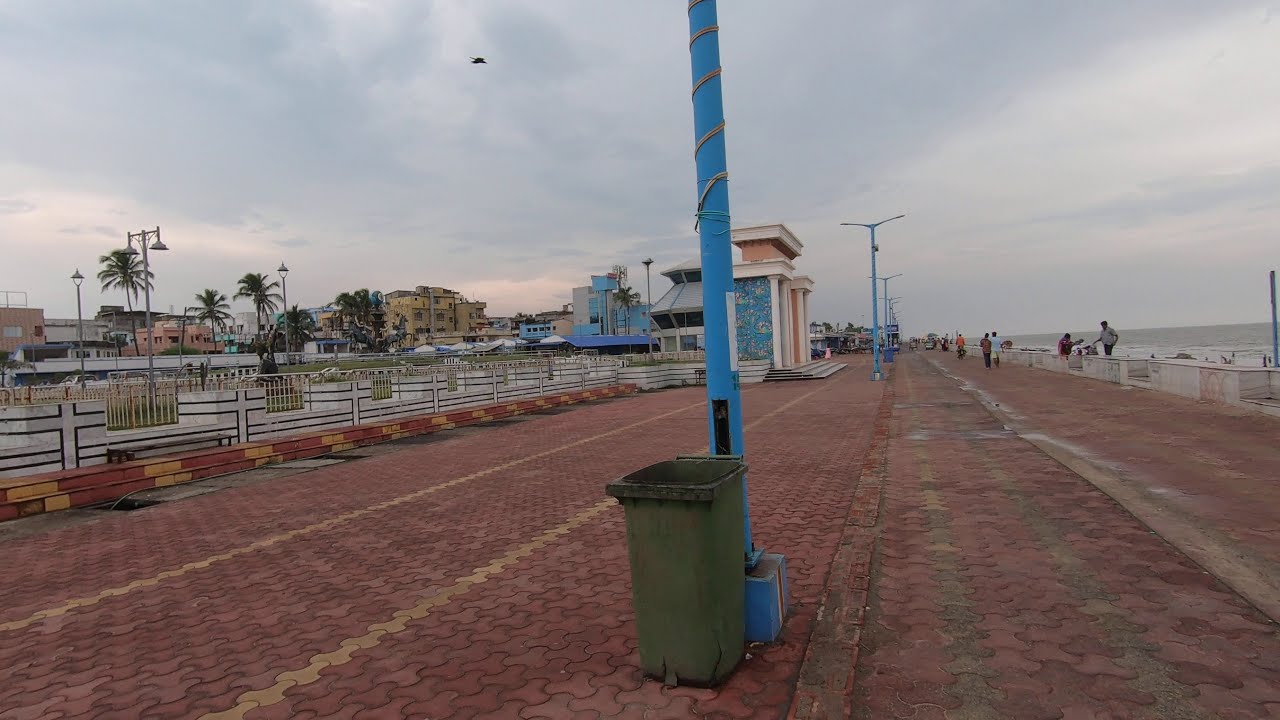The photograph depicts a large, open brick walkway beside a beach, likely located in Southern California or Florida. The expansive walkway, paved with red tiles, stretches from the foreground to the center background, interspersed with lines of yellow tiles on the left side and a gray drainage area. Prominently featured in the foreground is a grayish-green trash can next to a blue lamp post with string wrapped around its top half. Several more blue lamp posts are visible further along the walkway.

To the right, a short white wall borders the water, which occupies the rightmost part of the image. The left side of the walkway showcases a mix of buildings, painted in shades of red, yellow, and white, some appearing several stories tall. Slightly beyond these buildings, there seems to be a small structure adjacent to the walkway and possibly a train. The background is lively, with numerous people walking around, seemingly engaged in leisurely activities or shopping.

Overall, the scene captures a bustling coastal area with a broad, brick-paved promenade lined with distinctive blue lamp posts and various buildings.